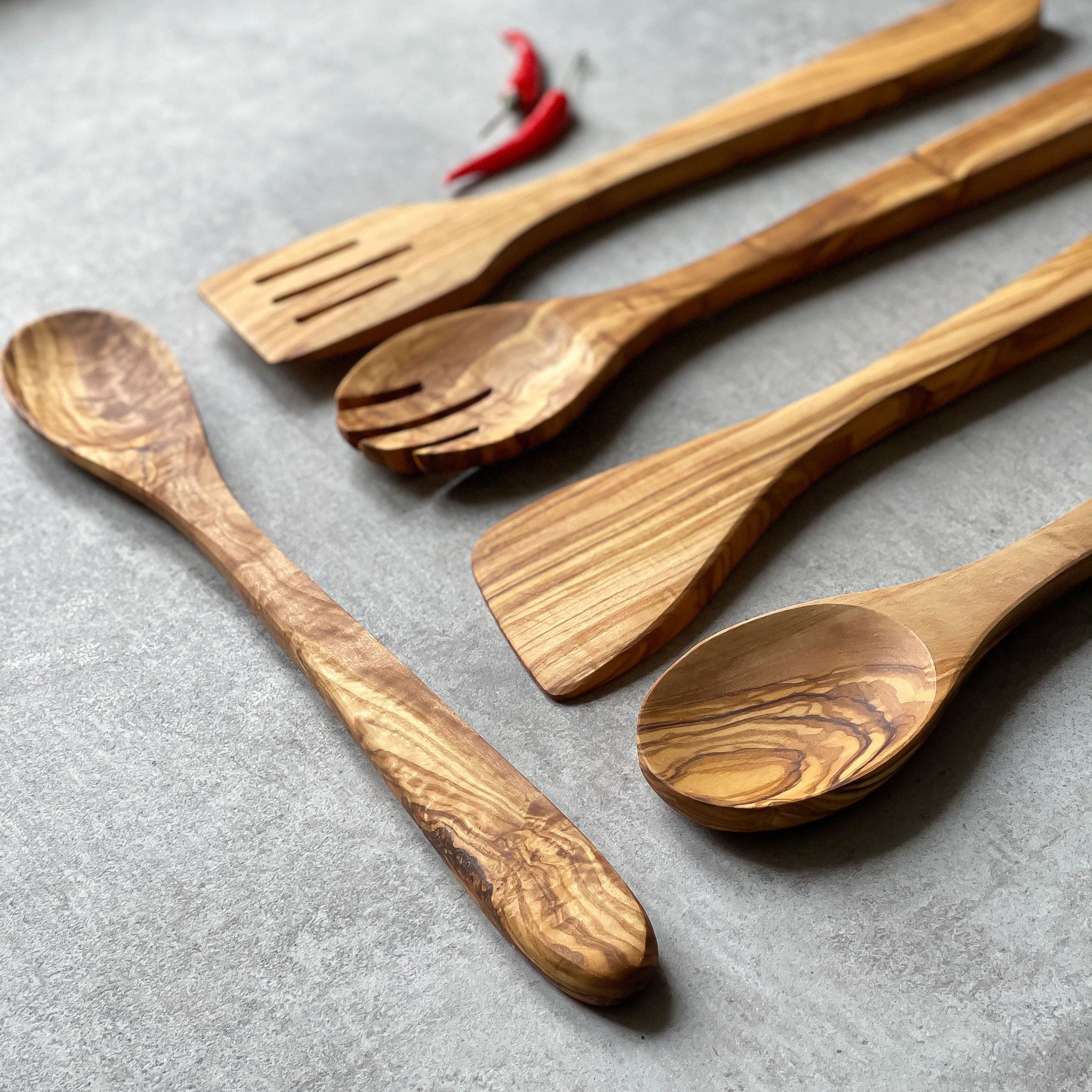This detailed photograph, taken in portrait mode, features a high-quality set of five wooden kitchen utensils laid out on a gray granite surface. The set comprises three wooden spoons and two spatulas, with one spoon and one spatula having grooves or slots cut into them. All five implements exhibit a natural wood grain with varying shades of brown, yellow, and tan, highlighting their sturdy, single-piece crafted construction. Arranged with four utensils pointing towards the lower left corner and one spoon pointing towards the top left, they create a balanced composition that enhances their visual appeal. The scene is completed by two vibrant red chili peppers with green stems positioned strategically above the wooden spatulas, adding a striking contrast. The primary colors in this minimalist image are brown, tan, red, and gray, emphasizing the earthy and rustic theme.